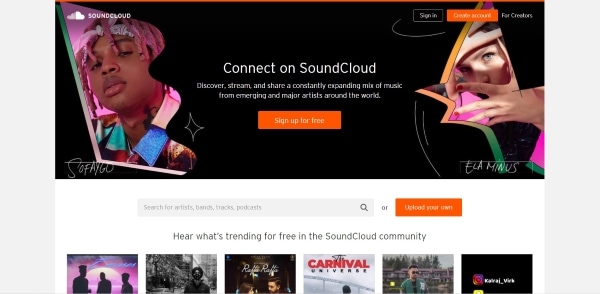This screenshot captures the homepage of a website with a sleek black background, prominently featuring a tagline in white text: "Connect on SoundCloud. Discover, stream, and share a constantly expanding mix of music from emerging and major artists around the world." Below this message, an inviting orange rectangle with white text encourages users to "Sign up for free."

On the left side of the screen, there is an image of a young man with striking pink braided hair, wearing a white bandana, and displaying a neck tattoo. To the right, a contrasting image features a woman covering her face with her hands.

At the top of the page, a black rectangle with white text offers a "Sign In" option. Below that, a search box invites users to "Search for artists, bands, tracks, or podcasts," accompanied by a magnifying glass icon. Adjacent to the search box, another orange rectangle with white text prompts users to "Upload your own."

Further down, the page highlights trending content in the SoundCloud community, signaled by the text "Here is what's trending for free in the SoundCloud community." Accompanying this section are various images, including one labeled "Carnival Universe" and another featuring a man wearing a green jacket and sunglasses.